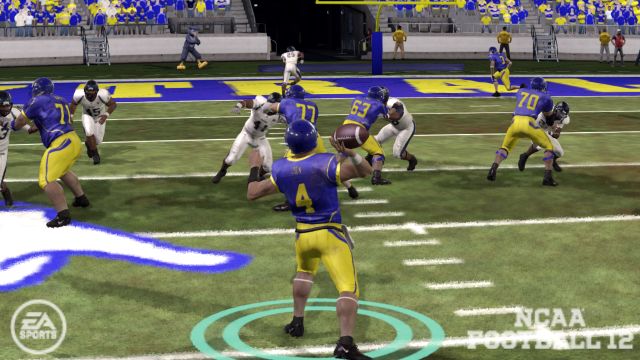The image depicts a vibrant scene from the computer game "NCAA Football 12" by EA Sports, as indicated by the EA Sports logo in a circle at the bottom left corner and the game title at the bottom right. The in-game action showcases two competing teams, one adorned in white uniforms with dark blue trims, and the other in blue and yellow gear. Central to the image is a player poised to throw a football, highlighted by two blue concentric circles around his feet, denoting his selected status. The stadium backdrop is filled with enthusiastic spectators predominantly dressed in blue and yellow, with a few sporting white attire. Notably, a blue bird mascot is visible, contributing to the lively atmosphere of the game.